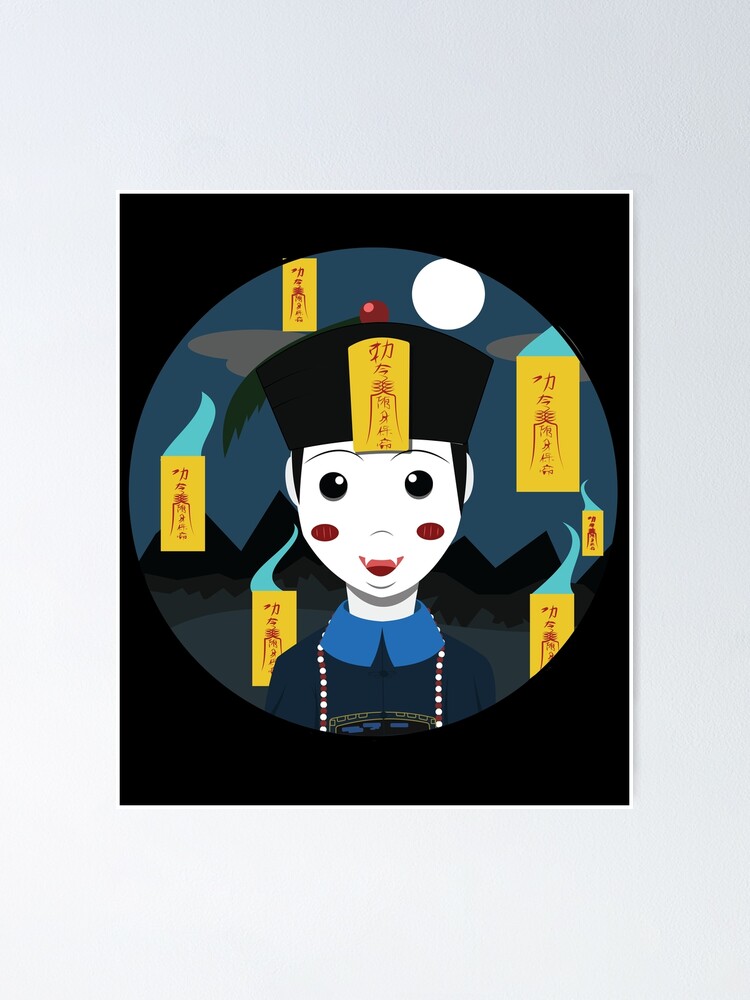This detailed description captures the essence of a vibrant and whimsical Asian-inspired painting. The image centers around a whimsical, animated portrait of an Asian man with strikingly white skin, accented by black circle eyes, red rosy cheeks, and a wide, fanged smile. His traditional black hat, adorned with a red bead at the top, displays a yellow ribbon bearing red Chinese text. He wears a dark blue shirt with a lighter blue collar and a white beaded necklace, suggesting a blend of traditional and possibly supernatural elements. Surrounding him are several yellow ribbons, also inscribed with Chinese characters, from which light blue wisps of smoke emanate. The backdrop features a night scene with a dark blue sky, gray clouds, and jagged, stylized mountains in silhouette. The image is framed in a black, circular shape with an off-white border, evoking a timeless, otherworldly feel, all under the watchful eye of a white moon.